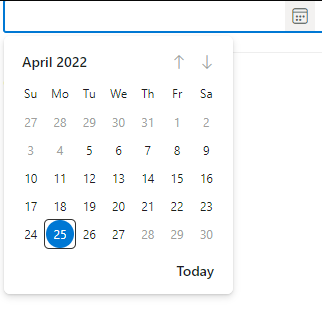The image depicts a minimalistic digital calendar view for April 2022. The plain calendar layout showcases all the dates in a grid format, with no specific dates highlighted or marked with events. The current date is the 25th, indicated by a blue circle around the number. On the bottom right, the word "Today" confirms the current day. The interface allows users to add events via a text field located near the top. Navigation capabilities include an arrow at the top and bottom, enabling users to scroll to previous or upcoming months, such as March or May. The overall design is straightforward with a white background and black digits, suggesting functionality over aesthetic embellishment. It remains unclear whether this calendar is a standalone application or integrated within another app.